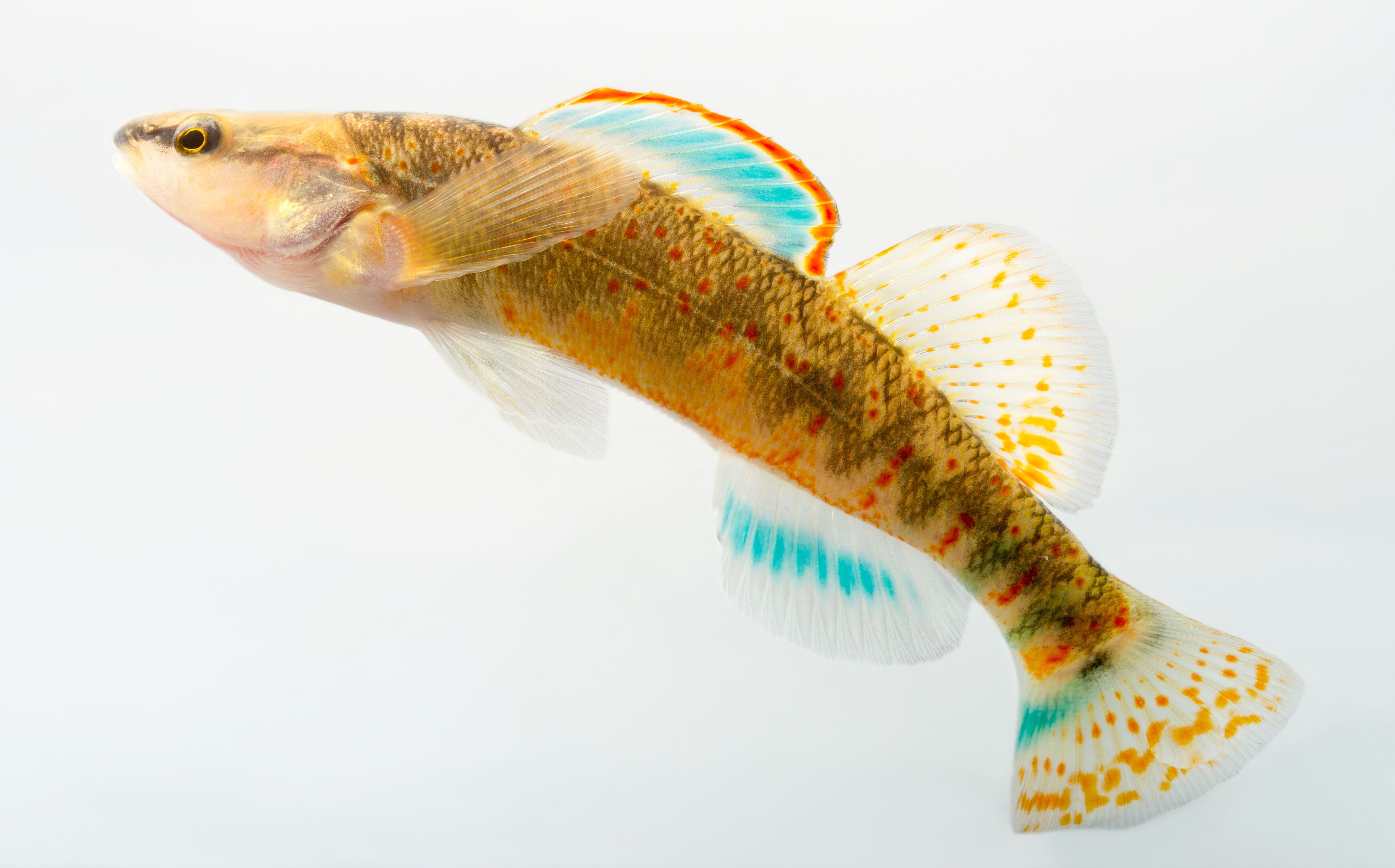This is a highly detailed, professional photograph of a small, colorful fish displayed against a grayish-white, translucent background. The fish, which appears to be around 2 to 3 inches long, boasts a complex pattern of coloration across its slim, elongated body. The eye is prominently black, bordered by yellow, and the fish's head shines with a glossy yellow and white iridescent sheen.

The body of the fish is primarily a mixture of yellow and white, adorned with zigzagging black lines and scattered orange-red dots, offering a vibrant mosaic of colors. Its fins are equally detailed: the top fin features light blue stripes edged in bright orange, while the subsequent fin displays a combination of white with yellow dots. Additionally, the fish has a fin near its bottom that mirrors the top fin’s light blue stripes, alongside side fins that are clear white.

Its tail fin continues the theme, presenting white with orangish-yellow dots and some blue highlights. The intricate interplay of these colors—white, yellow, black, red, orange, and teal blue—along with the checkered and spotted patterns, makes this fish a striking and vibrant subject. The perspective of the image offers a clear side view, devoid of any text or other distractions, focusing solely on the detailed and multi-hued beauty of the fish.